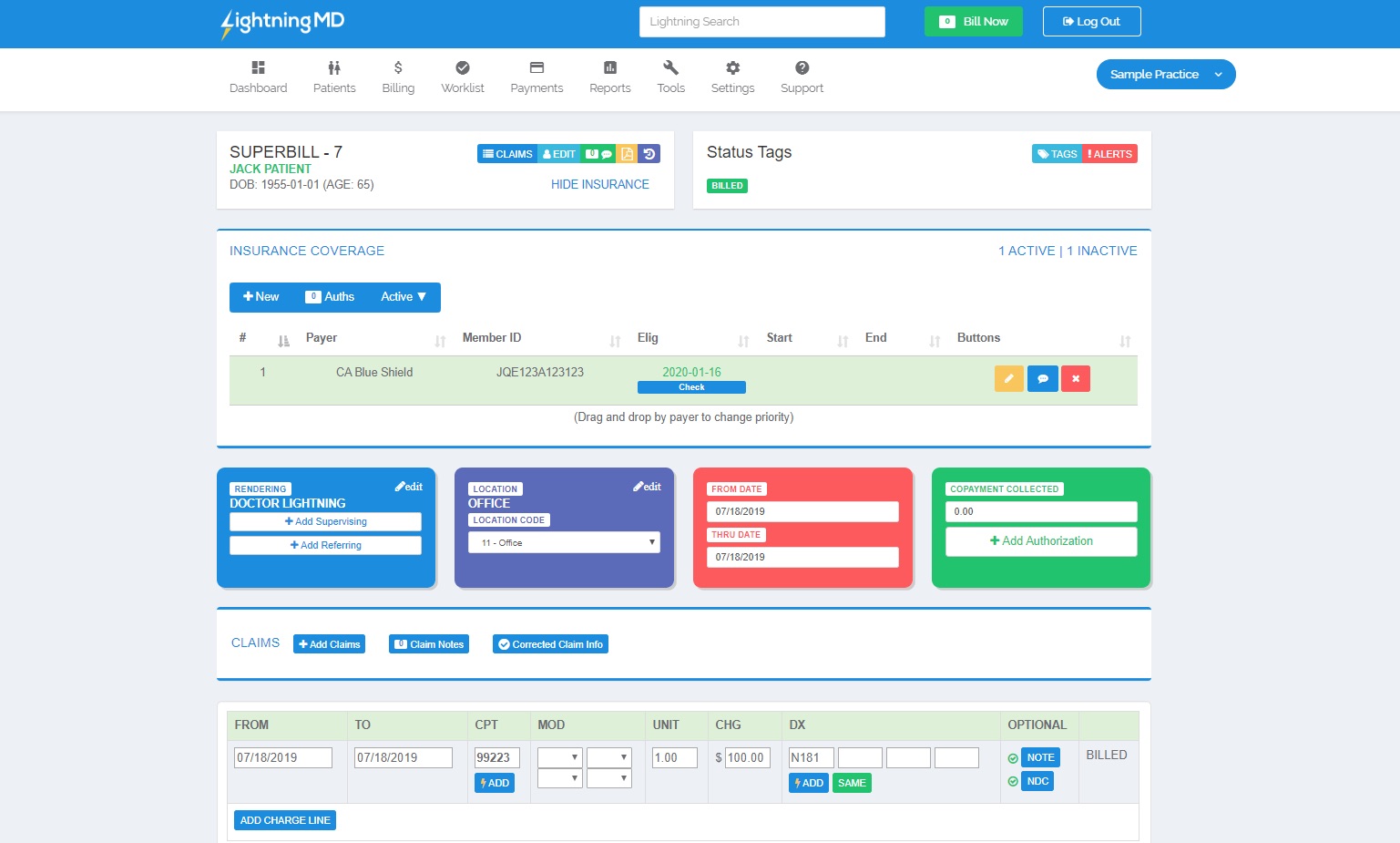The image depicts the homepage of the "Lightning MD" website. The standout feature of the design is the "L" in "Lightning," which is stylized to resemble a lightning bolt. At the top of the page, there is a thin blue navigation bar containing a lightning bolt-shaped search icon, a green button likely labeled with some action, and a logout button. Below this bar is a white navigation strip featuring various icons and buttons with labels. From left to right, these are: Dashboard, Patients, Billing, Work List, Payments, Reports, Tools, Settings, Support, and at the far end, a blue button with the white text "Sample Practice."

Further down, the page presents a form titled "Super Bill - 7" with an entry for "Jack Patient" and their date of birth. Adjacent features include colorful buttons that offer functions such as "Talk" and "Hide Insurance." Another section provides information about the patient's insurance coverage, specifying the payer as "CA Blue Shield."

Towards the bottom of the image, there are several color-coded informational windows: a blue window, a purple window, a red window, and a green window, each likely representing different categories or types of information.